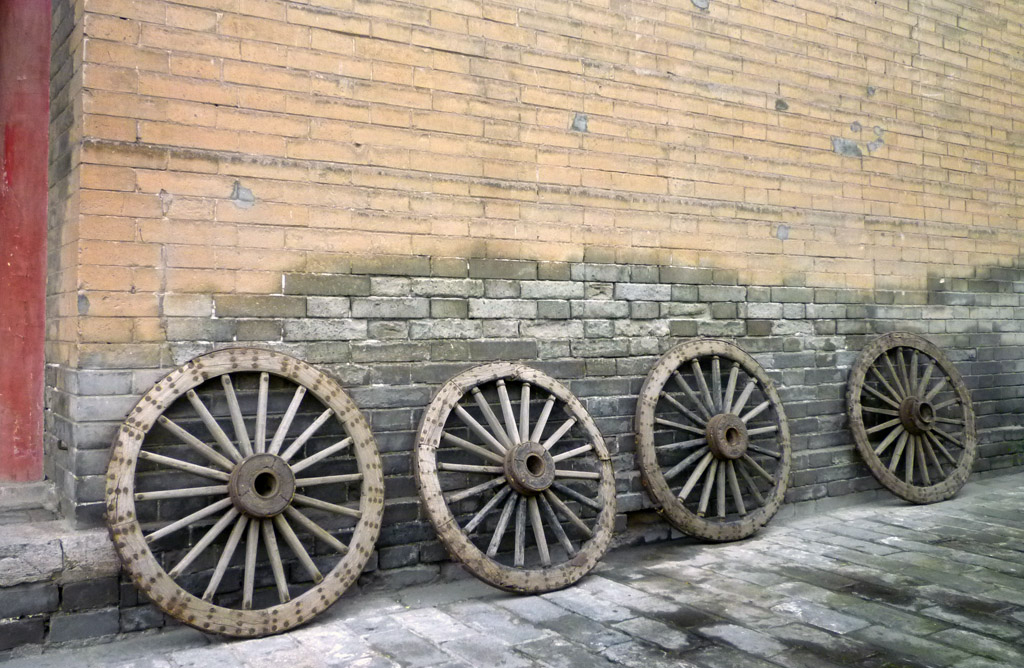This photograph captures the facade of an old brick building with a richly detailed, textured background and several historical elements. The building's upper portion features yellow and pale orange, faded paint revealing red bricks underneath, while the lower section showcases gray, weathered bricks. Leaning against this lower wall are four large, iconic wooden wagon wheels. These wheels, characterized by their light brown wood, are partially painted white, now peeling to reveal the natural wood color. The wheels have a metal center and are marked by spokes radiating from the middle. The ground below forms a cobblestone street that complements the overall vintage aesthetic. To the left of the image, a small, red door peeks into view, adding a final touch of historical charm.